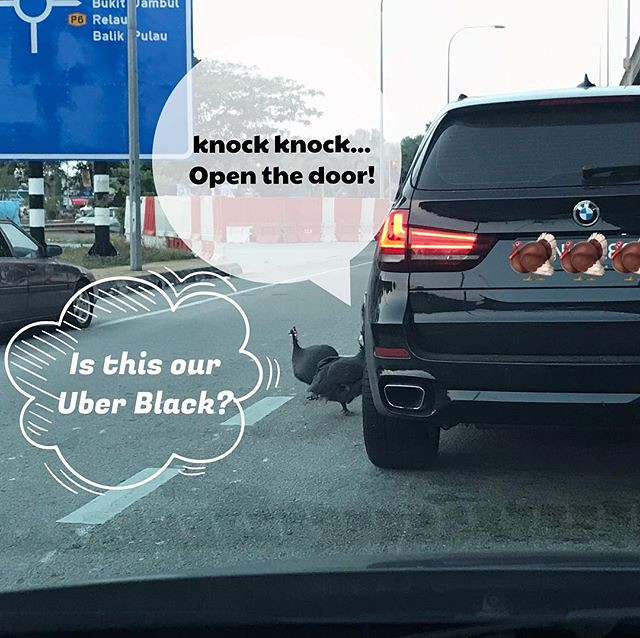The image is a humorous, staged photograph taken from inside a car, looking out toward the street. Dominating the scene to the right is a black BMW SUV with its brake lights on. The BMW's recognizable logo is clearly visible, and the rear of the car is adorned with three decals of turkey heads covering the license plate for privacy. Below the SUV, on the road, are two sizeable, dark gray birds, resembling fat pigeons or turkeys. These birds have comic-style speech bubbles, with one saying, "Is this our Uber Black?" in white print, and the other bubble reads, "Knock, knock, open the door." The setting appears to be in a city, with additional details such as a dark gray or black car on the left and a tall blue street sign that partially reads "r-a-t-a-u" and "be a l-i-k." The street itself is paved in light gray concrete with dotted white lines marking the lanes. Other elements visible include orange and white construction barriers in the background, street lights on poles, and an overcast sky.